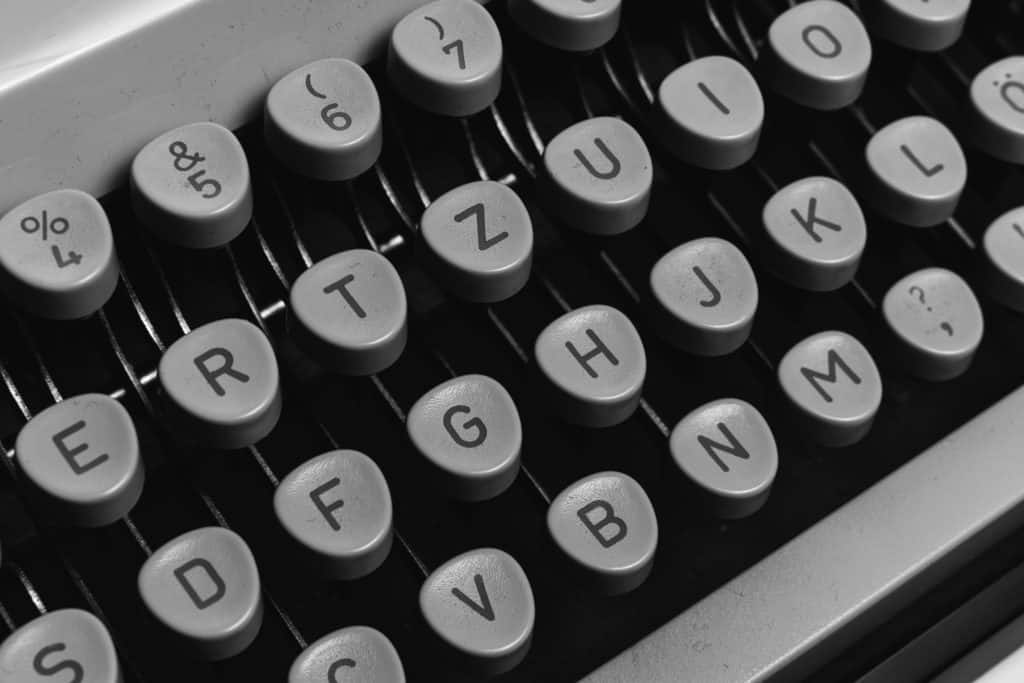A close-up, black-and-white photograph of an old-fashioned typewriter, showcasing the intricate details of its vintage keyboard. The typewriter's keys are prominently featured, arranged diagonally from left to right. The top row displays the number keys: 4 (%), 5 (&), 6 (left parenthesis), and 7 (right parenthesis). The next row consists of letters E, R, T, Z, U, I, and O. The subsequent row shows letters S, D, F, G, H, J, K, and L. The following row features letters V, B, N, M, along with a key showing a question mark above a comma. Additional details include the iron arms behind the keys and partial visibility of other keys, which are either half cut off or out of the frame. The typewriter itself has a gray finish and black lettering, with a spacebar visible at the bottom, anchoring the composition.